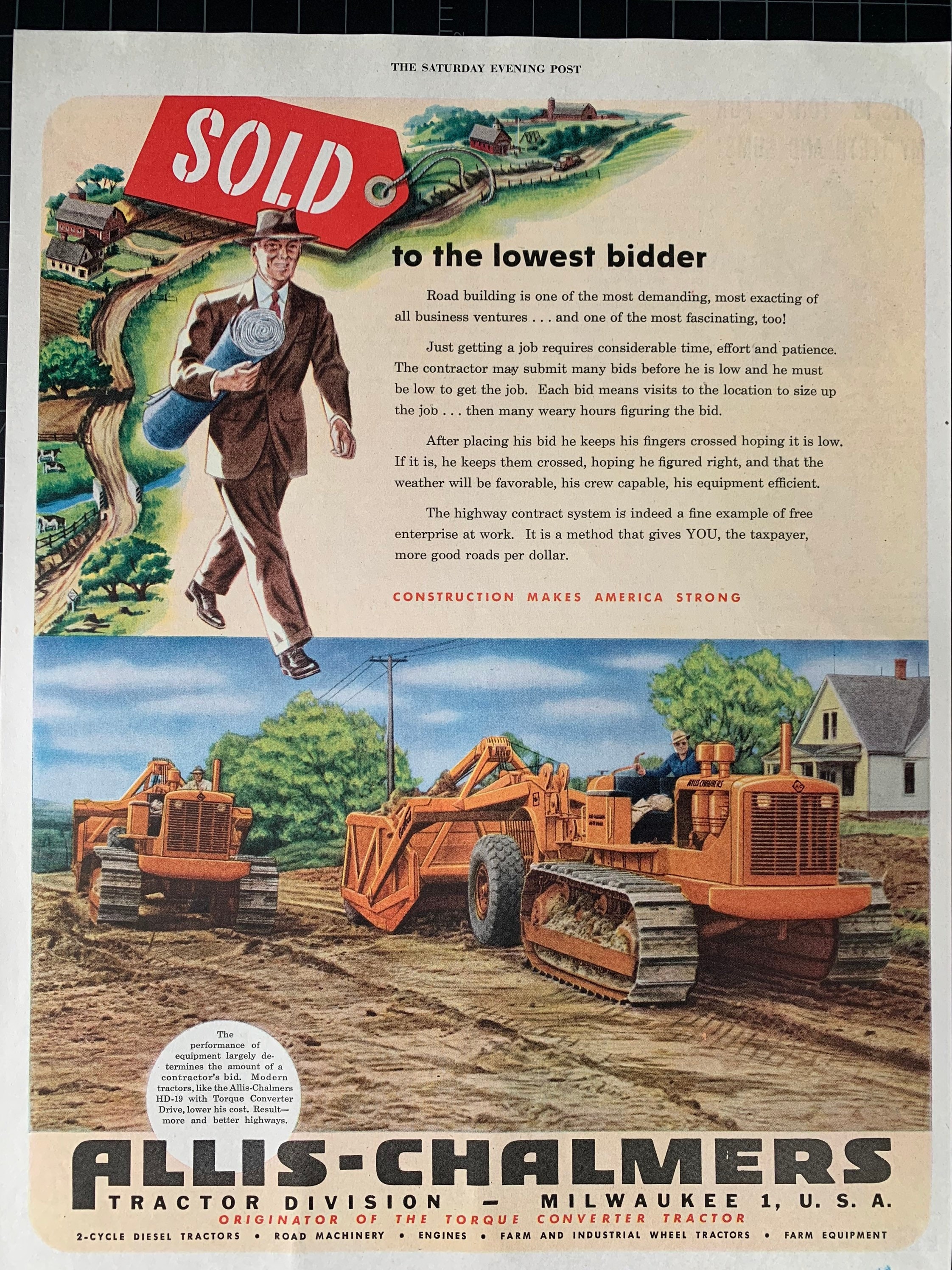The image is a vintage advertisement from the Saturday Evening Post, showcasing a drawing split into two parts. At the top, bold text reads, "Sold to the Lowest Bidder," accompanied by a detailed paragraph explaining the intricacies and challenges of the road-building industry, emphasizing the bid process' demands and the essence of free enterprise. Below this text, a salesman in a dated brown suit and hat is depicted walking with rolled-up plans, likely for a road system. A large red "Sold" sign is prominently displayed above his head, situated near a dirt road flanked by farmland, some houses, and trees under a blue sky populated with clouds. The lower part of the advertisement features an image of two orange caterpillar tractors from the Alice Chalmers Tractor Division, Milwaukee, USA. These tractors, navigated by drivers, are busy pushing dirt and grading the terrain, preparing for road construction, with power lines and an existing house visible in the background.